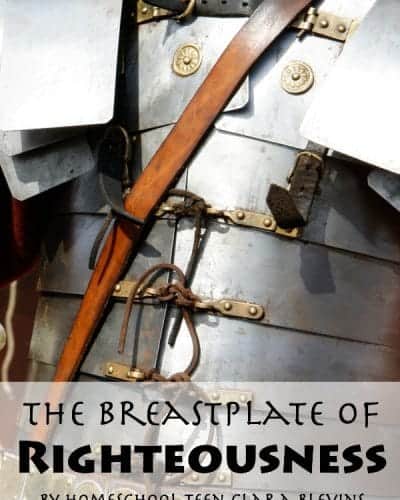The image appears to be the cover of a book titled "The Breastplate of Righteousness by homeschool teen Clara Blevins." The title, prominently displayed in bold capital letters on a white background at the lower third of the cover, emphasizes the word "righteousness." The central image features a detailed representation of a medieval-style metal breastplate. The breastplate itself is a silvery metal with ornamental gold buckles, buttons, and ties. A brown leather belt or sash runs diagonally from the left shoulder to the right hip, adding to the antique appearance. There are also shadows cast by the buckles, enhancing the depth of the design. The breastplate is adorned with various gold embellishments and features additional silver panels on the sides. The overall color scheme includes black, white, silver, gray, brown, and gold. The background of the cover is unclear, leaving the focus on the intricately detailed breastplate, evoking the appearance of old-fashioned armor worn into battle.